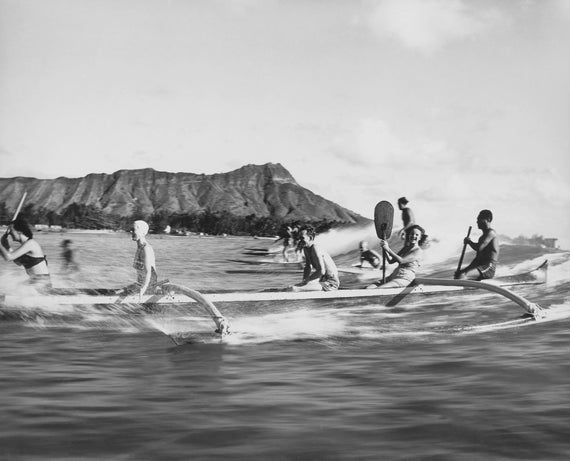This black-and-white photograph, likely from the 1950s, captures a lively scene set against a backdrop of a mountain ascending from the shoreline, possibly in Hawaii. The image features a long, narrow boat known as a catamaran, occupied by five people navigating the waters. The man in the back, dressed in a black swimsuit, appears to be paddling while looking into the distance. A woman behind him leans back and smiles, holding her paddle vertically. In front of her, a man leans forward, followed by two women; one wearing a bathing cap and another in a two-piece swimsuit, both actively paddling. The ocean stirs up small waves, adding a sense of motion to the picture. Surrounding the main vessel, several surfers and additional boats are visible, with some surfers catching waves in the background. The bright, almost clear sky featuring a few puffy clouds suggests it is daytime, and a line of trees before the mountain further enhances the scenic coastal setting.